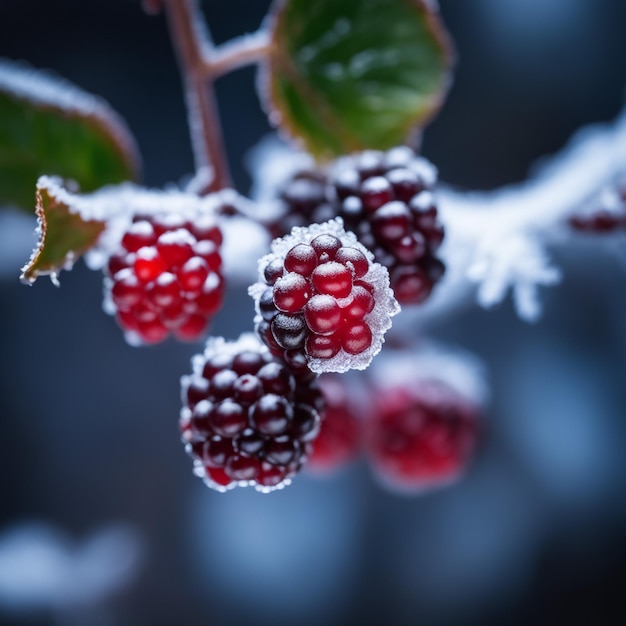This close-up image captures a small portion of a berry bush, showcasing a frosty cluster of berries against a blurred background with a bokeh effect. The focal point is a group of four berries, intricately detailed, covered in a light layer of frost. The berries display a range of colors from deep purple to reddish hues, highlighting the middle berry, which is heavily dusted with ice. Surrounding the berries, you can see green leaves with reddish veins, attached to a reddish stem also touched by frost. The background is a blend of blackish, grayish, and bluish tones, enhancing the sharp, cold atmosphere of the scene.